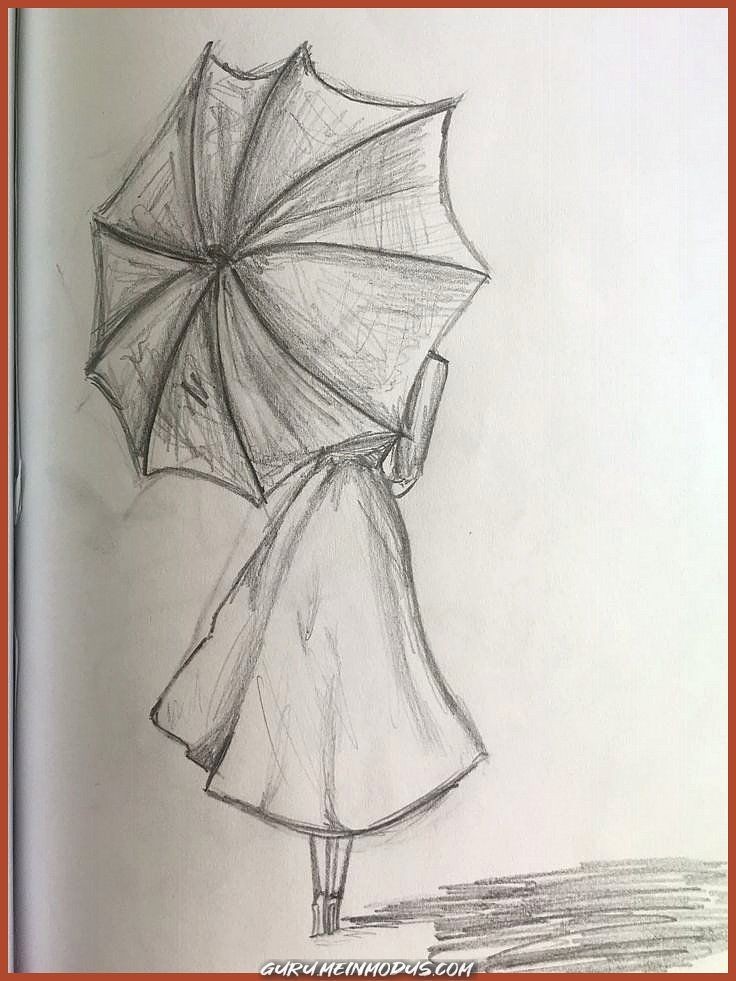The image showcases an exquisitely detailed pencil or charcoal drawing, prominently featuring the upper left-hand side. Here, the artist has skillfully rendered the back of an umbrella, utilizing remarkable shading techniques to create a realistic effect. Carrying the umbrella is a woman, visible from the back, adorned in a beautifully detailed 1950s-style circle skirt. The shading on her skirt is particularly commendable, demonstrating the artist's talent. The woman's legs are positioned very closely together, almost appearing as a single leg. A hint of her right shoulder and forearm, clad in a long-sleeved shirt, is also visible. At the bottom right-hand corner, subtle shading suggests the ground, while at the very bottom, the artist's name is inscribed, though it is unfortunately too small to read.